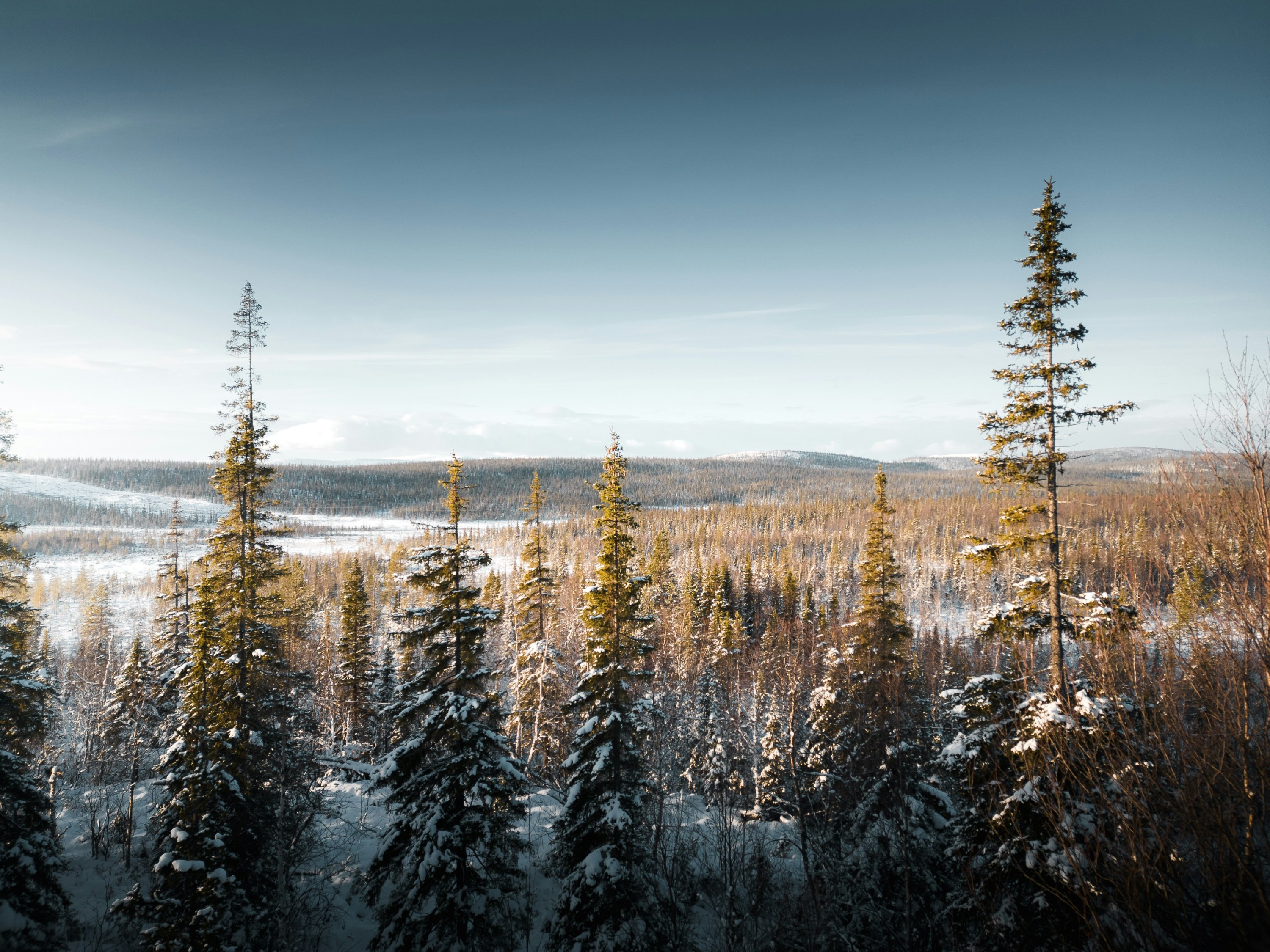This horizontally oriented outdoor photograph captures a breathtaking view from a ridgeline, showcasing a vast and undulating mountainous valley densely covered with evergreen pine trees, many of which have a light dusting of snow. Some of the trees in the foreground, particularly four prominent ones to the left and a tall tree accompanied by a bush to the right of center, exhibit green foliage sparsely dusted with snow, while others show branches devoid of needles and foliage, indicative of seasonal changes. The snowy tree line stretches deep into the distance, blending with the brownish-green hues of the middle ground and gradually disappearing into the slightly hilly horizon. Beyond the horizon, the sky transitions from a white and grayish hue at the skyline to a darker blue as it ascends, streaked with thin, wispy clouds. Though sunlight bathes the landscape, the sun itself remains out of the frame, subtly illuminating the scene from the right, enhancing the varying shades of blue and green that dominate the image.